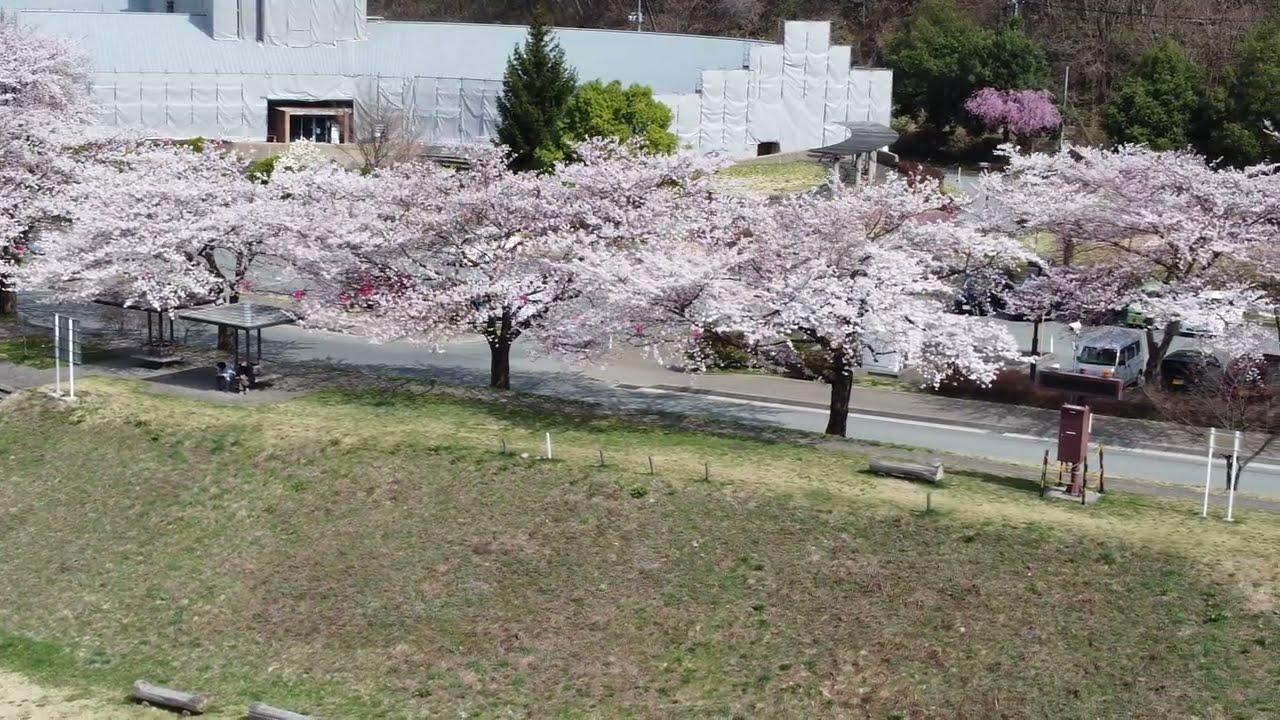This image, taken outside on a bright sunny day, captures a picturesque landscape. The lower portion, starting from about the left center and diagonally descending towards the lower right corner, features a gently sloping hillside covered with a mix of thin green grass, brown patches, and dirt. Crowning the hill are rows of cherry blossom trees with dark stalks and long branches adorned with vibrant pink and white flowers.

At the hill's crest, a line of stakes suggests the remnants of a former fence. Beyond this, a paved two-lane road runs, bordered on both sides by additional rows of blooming cherry blossom trees. Tucked among these trees is a push cart, and a person stands beside it. A white van is parked nearby.

In the upper left background, a large white building appears to be under construction, draped in weather-protective coverings resembling scaffolding with white tarps. The scene is further animated by people relaxing under small canopied benches near the road, and several cars are visible in a parking area beyond. This blend of natural beauty and scattered human activity creates a tranquil yet vibrant snapshot of the day.